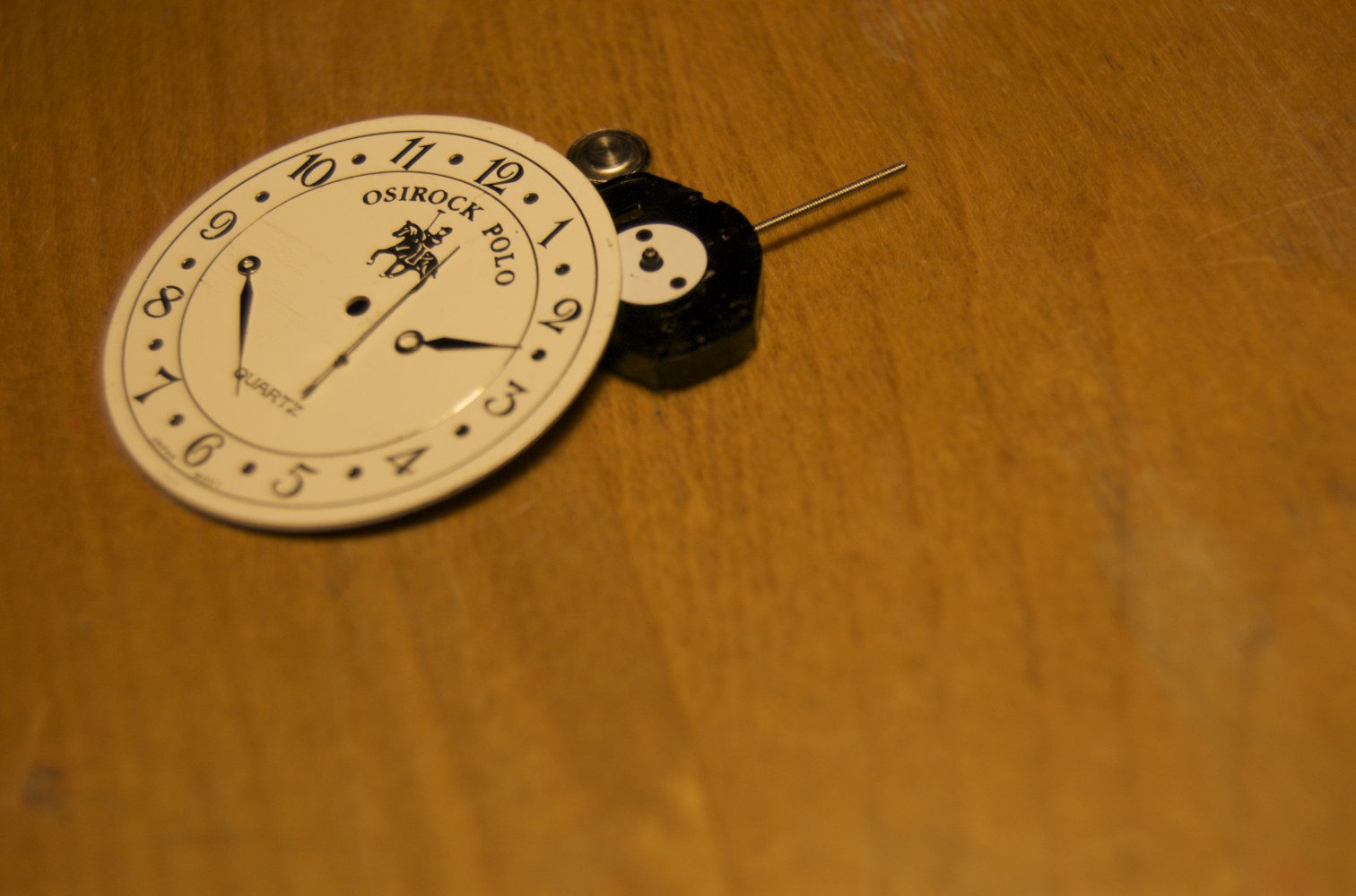The photograph showcases a close-up view taken on a wood grain table, with a wide and tall frame. Dominating the top left quadrant of the image, approximately 30-40% of the frame, is a partial view of an Aussie Rock Polio brand quartz watch. The face of the watch is distinctive, featuring a vintage design with ornate numerical markings from 1 to 12, interspersed with small dots.

The image captures the watch face angled slightly upward to the left, providing a clear view of its intricate details. At the center of the watch face, there is an illustration of a polo player mounted on a horse, energetically raising a polo stick as both rider and horse move sideways, adding a sense of motion to the image. 

The watch hands appear somewhat disordered: the larger hand points towards the bottom right, the smaller hand towards the top left, and the second hand is aligned with the 12 o'clock mark. Attached to the backside of the watch face is a small black plastic nub with a white center disc, likely serving as a connection point to the watch mechanism.

In the background, components like a battery or a gear are faintly visible, positioned north of the connecting nub. Extending upwards towards the top right of the frame is the watch rod, hinting at its mechanical complexity. While the majority of the watch's structure is absent, the detailed close-up of the face and internal components offers insight into the watch's elaborate design.